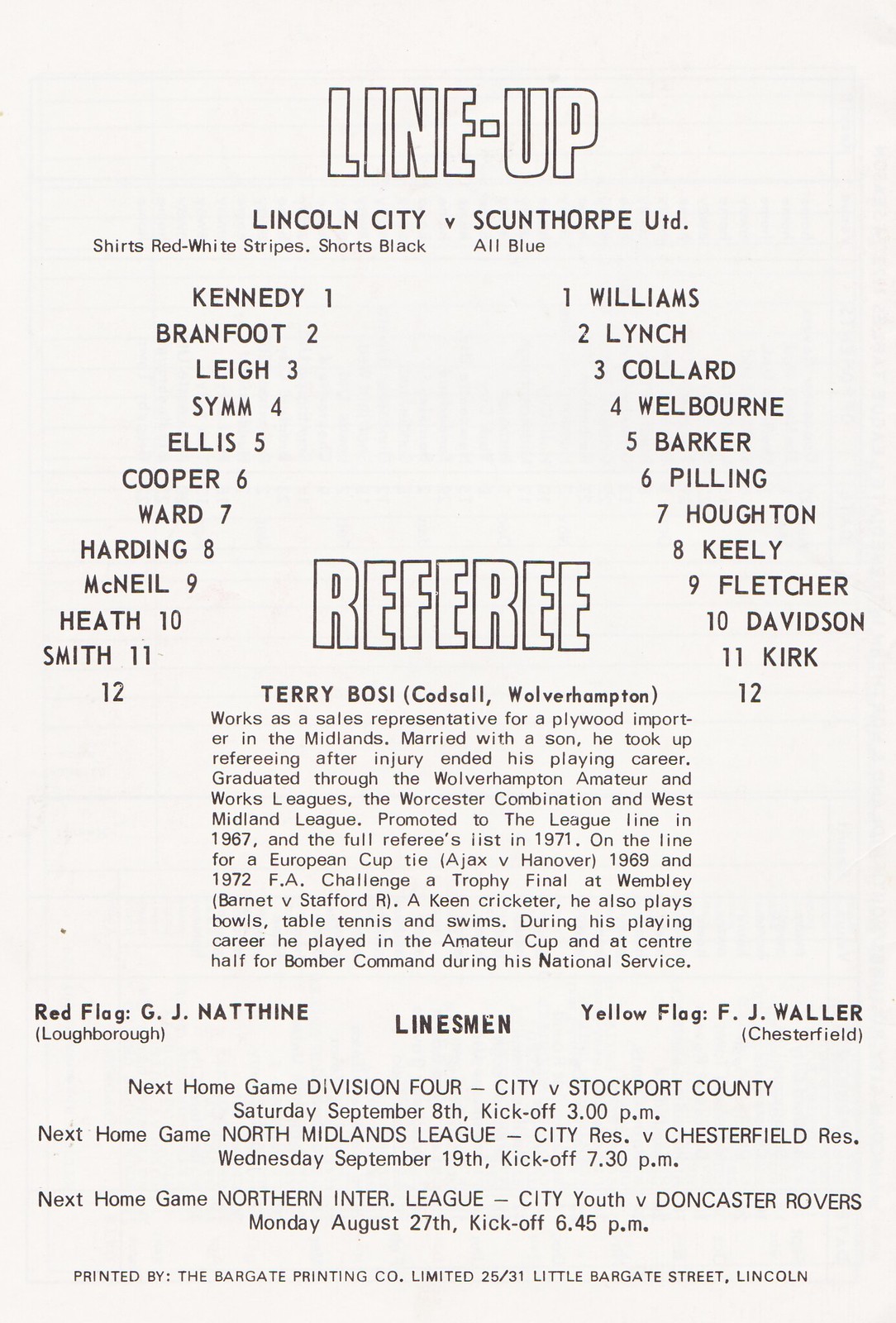This vertically aligned rectangular black and white print page, likely created on a computer and printed on slightly off-white cardstock, prominently features the word "LINEUP" at the top in block letters. Below, the lineups for Lincoln City and Scunthorpe United are presented. Lincoln City is described with red and white striped shirts and black shorts, with player names and numbers listed from 1 to 11, and the 12th slot left blank. Scunthorpe United, depicted in all blue, follows a similar format with their players listed from 1 to 11, also leaving the 12th spot blank. Centralized large block letters announce the referee, Terry Boese from Codsall, Wolverhampton, accompanied by a justified paragraph detailing his biography. At the bottom, details include the names and origins of the assistant officials: G.J. Nathine as the red flag official, and F.J. Waller from Chesterfield as the yellow flag official. Additionally, the page provides the names and locations of the linesmen, alongside a list of upcoming games.